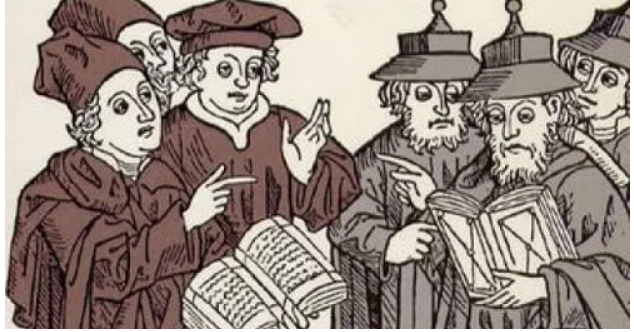The image portrays a detailed artist's rendition, featuring two groups of people, each consisting of three individuals, facing each other in what appears to be a heated debate. On the left, the group of three is dressed in red long-sleeved, loose-fitting dresses and red berets. They are pointing towards the other group, and one person is prominently holding a book. The right group is adorned in grey long-sleeved, loose-fitting dresses with unique caps resembling domes that extend over their foreheads, topped with a ball-like structure. This group also has a member holding a book, mirroring the gesture of the group on the left. The setting of the image is black and white with sepia tones, suggesting an aged or historical feel. The attire and books suggest that the figures may be related to a religious or scholarly context, possibly monks or priests, involved in a theological or philosophical dispute. The intricate details of their attire and expressive hand gestures underscore the intensity of their interaction.